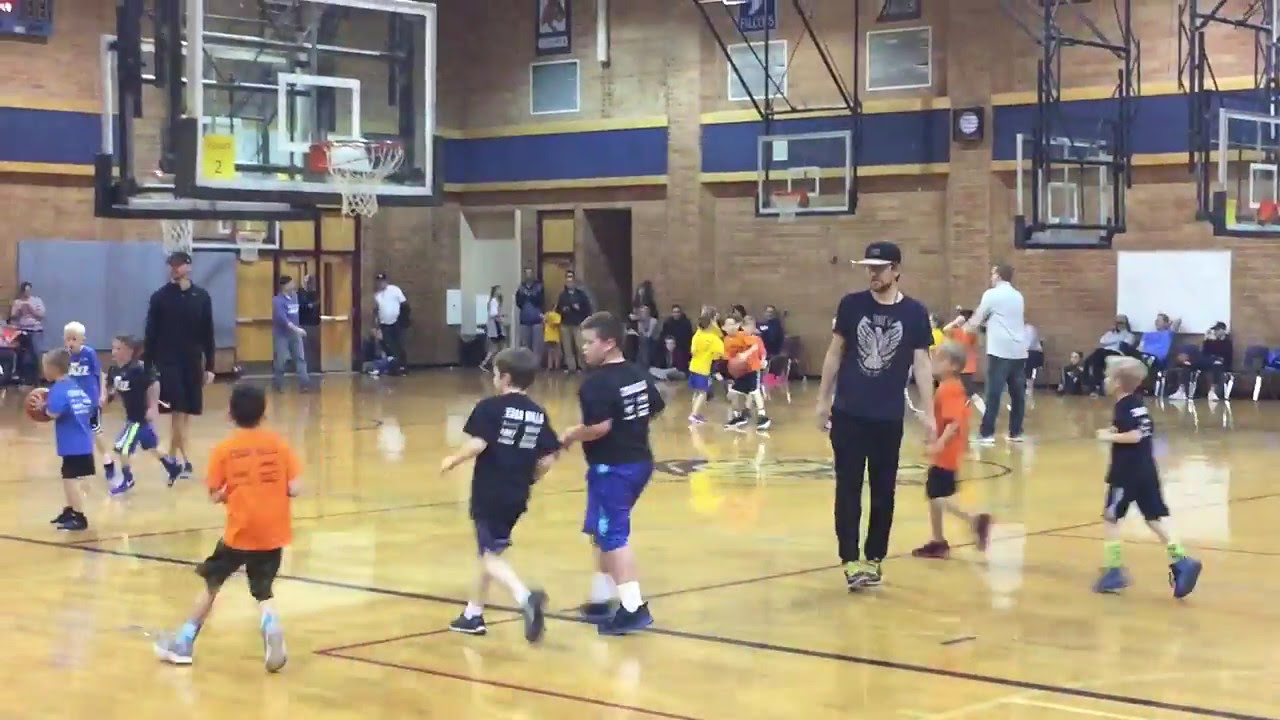In this image, a vibrant scene unfolds within a school gymnasium, featuring a glossy, lacquered hardwood floor marked with paint lines and a team logo. The basketball court, centered in the photo, hosts about 12 young players dressed in multicolored t-shirts—orange, black, blue, and yellow—indicating a practice session rather than an actual game. Basketball hoops with clear backboards hang from the ceiling, totaling five in number. Amidst the action, a taller man in a t-shirt and hat, possibly a coach with a whistle around his neck, stands out, guiding the players. The gymnasium's brick walls are adorned with posters and a white notice board, and the color scheme includes shades of cream, blue, and yellow. Wooden double doors and plastic chairs with people, likely parents and additional coaches, are visible in the background, contributing to the bustling atmosphere of this indoor basketball practice session.